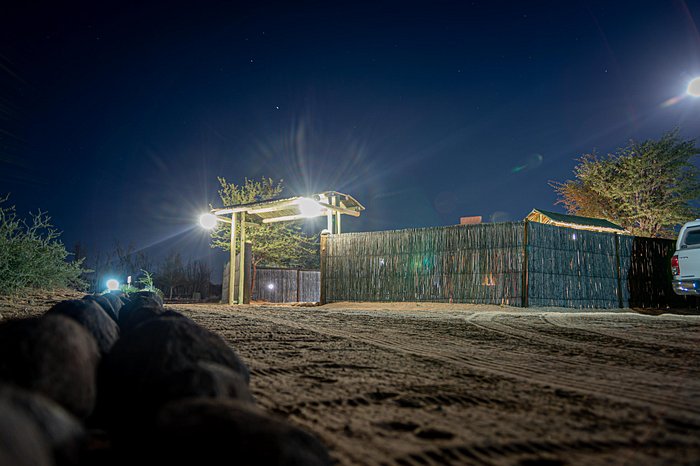The nighttime HDR photograph captures a secluded, wooded area centered around an enclosure made of a rustic, possibly bamboo or twig-like fence arranged in an L-shape. The image, taken from ground level, shows dirt in the foreground and a partially visible black object to the left. At the center of the photograph stands an archway or gateway reminiscent of a pergola or entrance for vehicles, adorned with two intensely bright lights. Behind this structure is a tall tree, while another bright light shines distantly on the left and an additional one glows above a tree on the right, partially illuminating the back of a white SUV or truck. The dark blue sky is speckled with a few stars, adding a serene contrast to the vivid artificial lights dominating the scene.